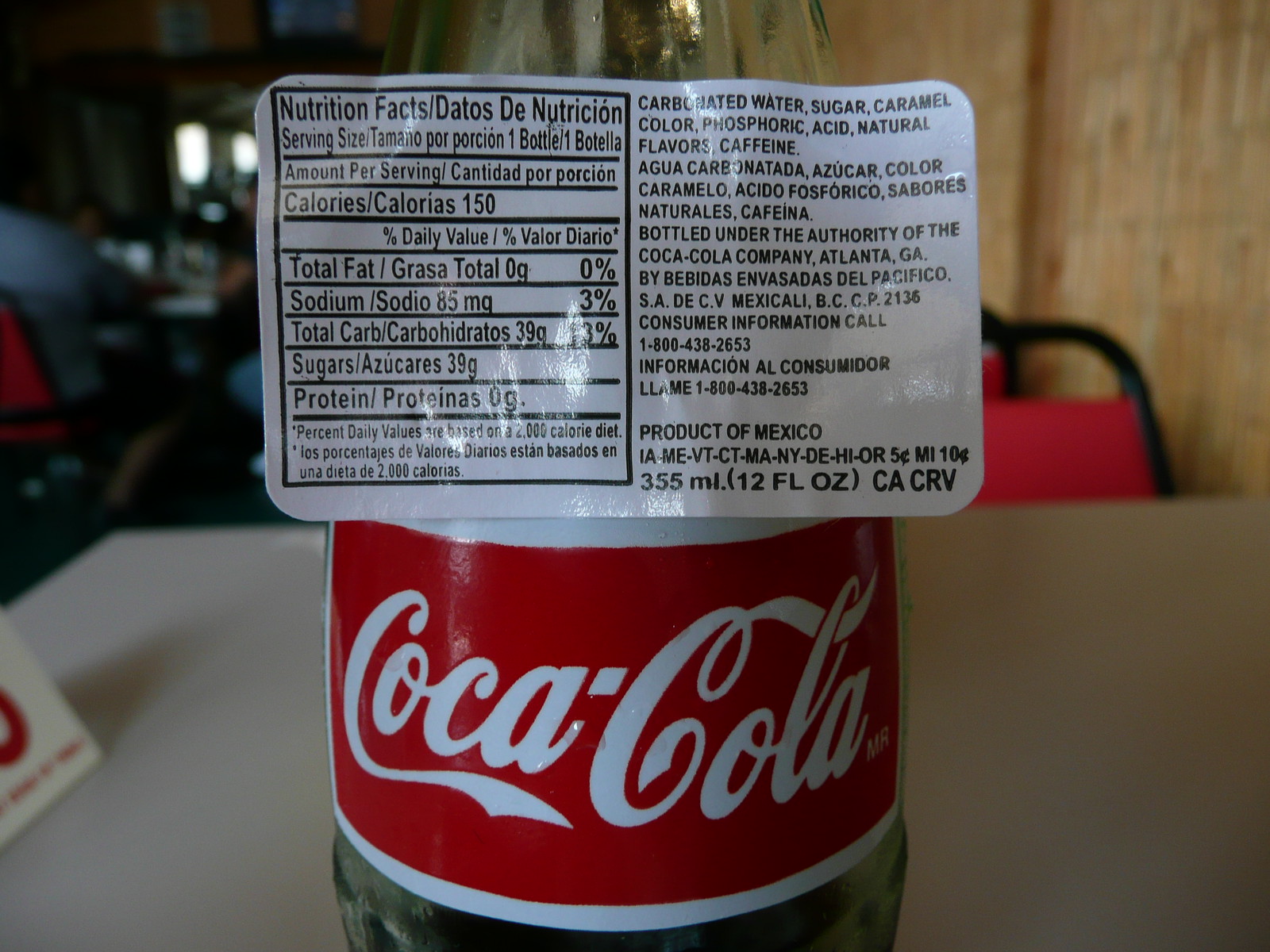A clear Coca-Cola bottle is prominently displayed in the center of the image. The iconic red label with "Coca-Cola" written in white letters, trimmed in white, adds to the classic look. This label, partially peeled off the bottle, is also placed in the foreground of the picture, showcasing the "Nutrition Facts" panel. The white label with black text details various nutritional information per serving: 150 calories, 0g total fat, 85mg sodium, 39g total carbs, 39g sugars, and 0g protein. Additional text beneath outlines that percent daily values are based on a 2,000-calorie diet and lists the ingredients: carbonated water, sugar, caramel color, phosphoric acid, natural flavors, and caffeine. There is also information in a different language, contact details for consumer information (1-800-438-2653), and a note stating it's a product of Mexico containing 12 fluid ounces. The bottle rests on a beige countertop, with a backdrop featuring a brown wooden wall, a red chair trimmed in black, and a muted background on the left side, adding context and setting to the image.